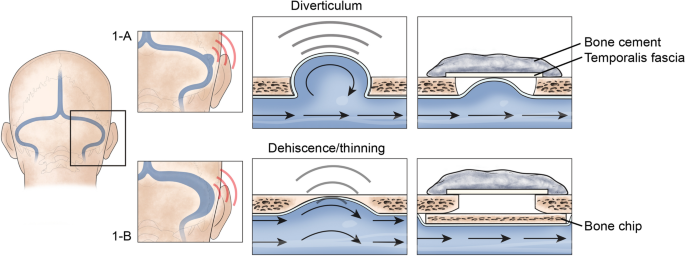The image features a detailed medical diagram focused on the back of a human head, illustrating a blue pathway extending between the ears and up the center of the head. On the left, a drawing of the back of the head is displayed, while on the top and bottom are labeled close-up diagrams: 1A and 1B. Diagram 1A depicts red waves emanating from the right ear and highlights terms like "diverticulum" and "bone cement into porous fascia," with arrows suggesting the pathway of bone cement. Diagram 1B shows a larger vein or pathway labeled "dehiscence/thinning," accompanied by different wave patterns and the mention of a "bone chip," indicating some medical intervention or abnormality in this version. Both diagrams employ black arrows to emphasize specific areas and changes between the images, illustrating a comparative view of the conditions depicted.